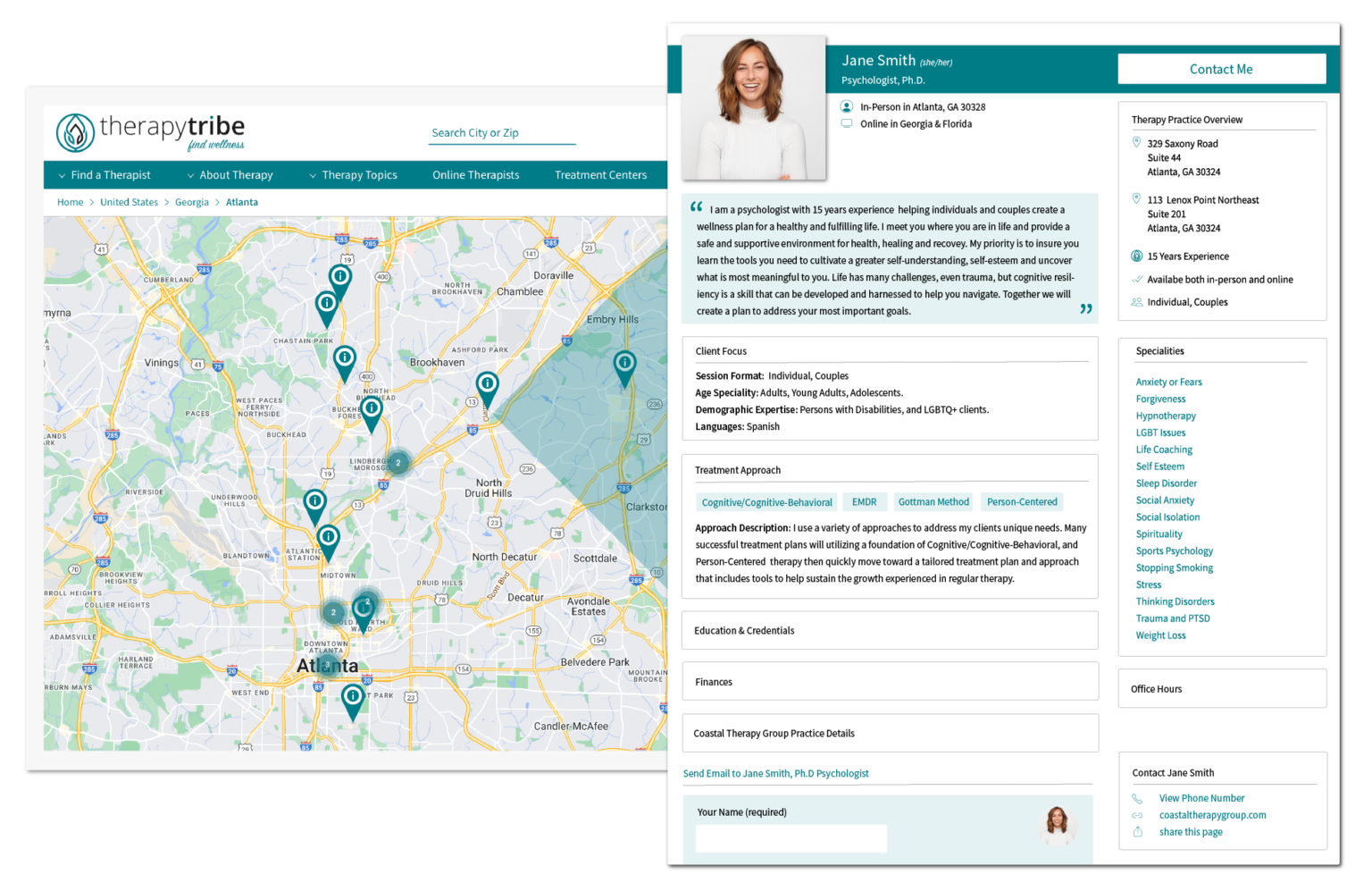**Detailed Caption:**

This composite image consists of two screenshots from the Therapy Tribe website. On the left-hand side, the main page is partially visible, featuring a background photo of a world map adorned with pinpoint markers indicating various locations, potentially places where one can find therapy services. At the very top, the website's logo, "Therapy Tribe," is prominently displayed in turquoise. To the right of the logo, there's an input field labeled "Search City or Zip," accompanied by several dropdown menus for easy navigation. Below these elements, a turquoise banner appears, though the text within it is not readable.

On the right-hand side of the image, an overlay page centers around a therapist named Jane Smith. A professional headshot of Jane Smith is shown to the right of the overlay. Adjacent to her photo, a striking white box with "Contact Me" written in turquoise invites visitors to reach out. While the smaller text is not legible, it is inferred to contain details about Jane Smith's qualifications, specialties, and possibly her location. This section includes an option to call or contact Jane Smith directly, underscoring her availability for therapy services.